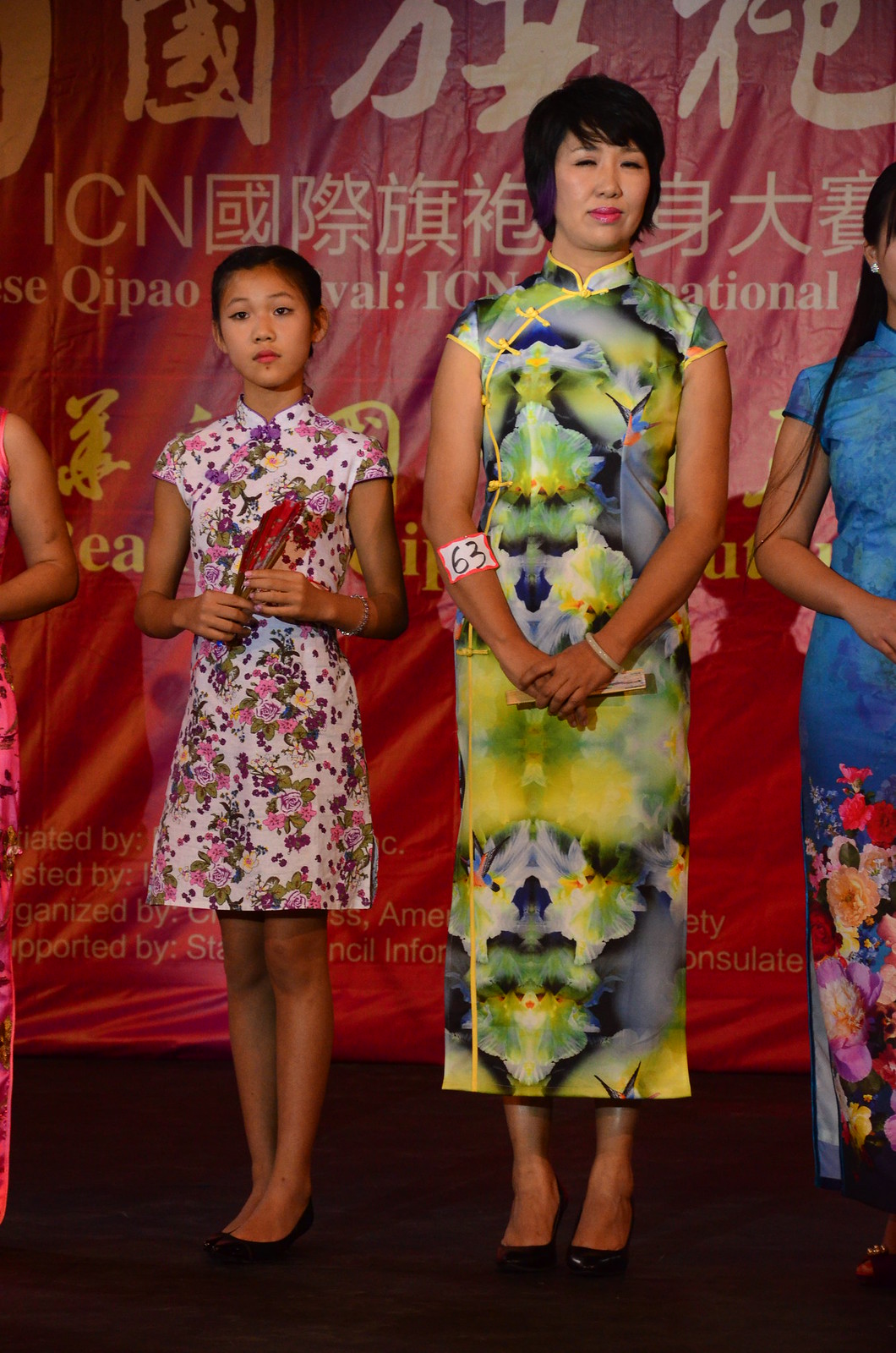The photograph captures a scene on an indoor stage featuring four individuals, though only two are fully visible in the center. The two people who are prominently visible include a young girl and an adult woman, both of Chinese ethnicity. The girl, approximately 11 or 12 years old, stands to the left, dressed in a vibrant white dress adorned with colorful floral patterns, and holding a red fan. She is wearing black shoes. To her right stands an adult woman, likely in her 30s, with short black hair. She is dressed in an A-line dress featuring blue, green, and yellow hues in what appears to be a floral pattern, and she has a tag on her left arm marked with the number 63. The stage floor is black, and behind them stretches a large red banner with text in both Chinese and English, further hinting at the cultural context of the setting. On the far edges of the image, only parts of two other individuals are visible: to the woman's right, a woman in a long blue dress with floral patterns, and to the girl's left, an arm of another person.